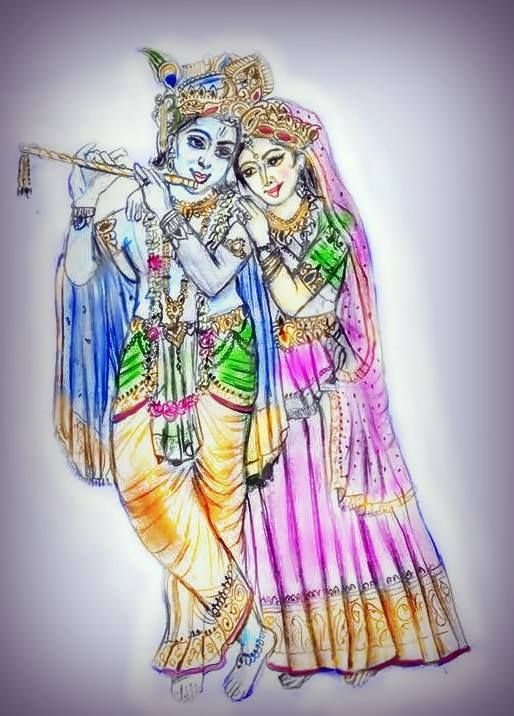This image portrays a colorful and vivid painting, possibly executed in watercolor or crayon on a white background with a smoky purplish-black outline. Central to the composition are two individuals in ornate, gypsy-like attire, each with intricate headdresses embellished with blue, green, red, and gold colors.

The person on the left, whose gender is ambiguous, is likely male, and is depicted playing a yellow flute adorned with dangling ornaments. He dons a blue cloak, brown pants with green accents, and a green belt trimmed in gold. His headdress is a gold crown with blue, yellow, and green detailing. He is barefoot, with henna tattoos on his forearms and wrists, and is wearing numerous necklaces and armbands.

The person on the right, who seems female, is dressed in a colorful ensemble featuring a pink, red, and yellow cape, a pink dress with gold trim, green arm sleeves, and a pink scarf with black dots. She also wears an elaborate gold headpiece with red stones. Like the other individual, she is barefoot and adorned with henna tattoos, necklaces, and armbands. The two figures are smiling, leaning their heads together, with the woman on the right affectionately leaning on the person playing the flute. Their clothing and accessories are richly detailed, with belts and embellishments at the hips, enhancing the vibrant, gypsy-like aesthetic of the scene.